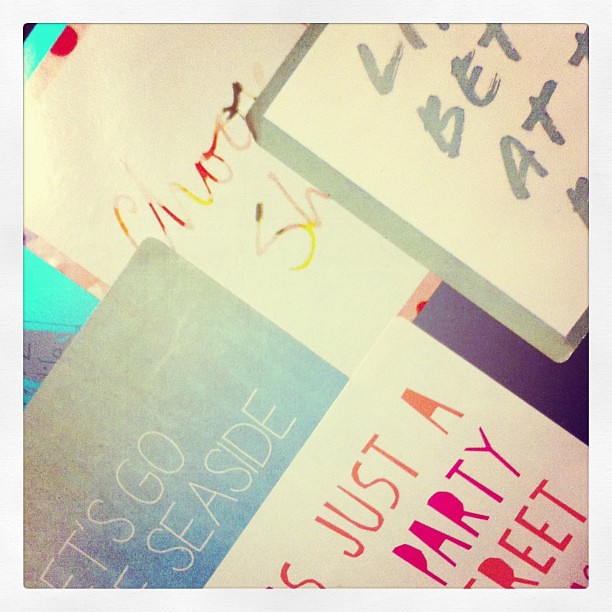The image is a high-exposure, washed-out collage of various cropped logos and signs with an eclectic mix of fonts, including cursive and printed styles. The logos are stacked on top of each other, creating a chaotic yet intriguing pattern. Dominant colors include shades of pink, orange, yellow, red, and gray. Key visible texts include "Let's Go Seaside" on a grayish background with white letters, "jesta party" with an orange and pink font on a white background, and partial letters like "L, B, and A" and "R-E-E-T," possibly from the word "street," in a mixture of orange and purple. The logos appear to be on square signs with rounded edges, though none are fully legible. The overall aesthetic suggests a collage of greeting cards or promotional signs with overlapping and fragmented text.